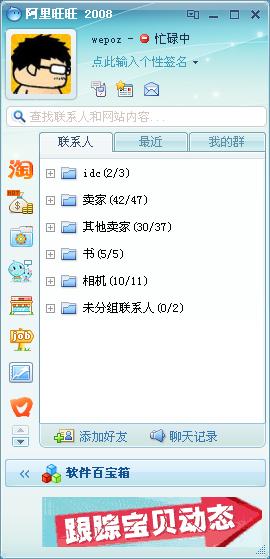The image depicts a screenshot from a smartphone, featuring a UI in either Japanese or Chinese characters. The dominant colors are light blue and white, with darker blue highlighting certain sections. In the upper left corner, there's an avatar of a cartoon boy with black spiky hair, rectangular glasses, and a sparse mustache, facing sideways. Next to the avatar is the username "WEPOZ" and the year "2008" is displayed above. Below the avatar, there's a search bar followed by a tab listing six blue folders with various labels, one reading "IDK 2 out of 3". On the left side, there are several navigational icons for different categories: a Japanese letter, currency symbol, a camera, a friends list, a store, job listings, and a graph. Additionally, a large red arrow points to the right at the bottom. The screen also contains battery and notification indicators, as well as an X button for closing. The overall layout suggests the interface is designed for comprehensive organization, possibly involving chat or communication tools, banking, and job-related functions.